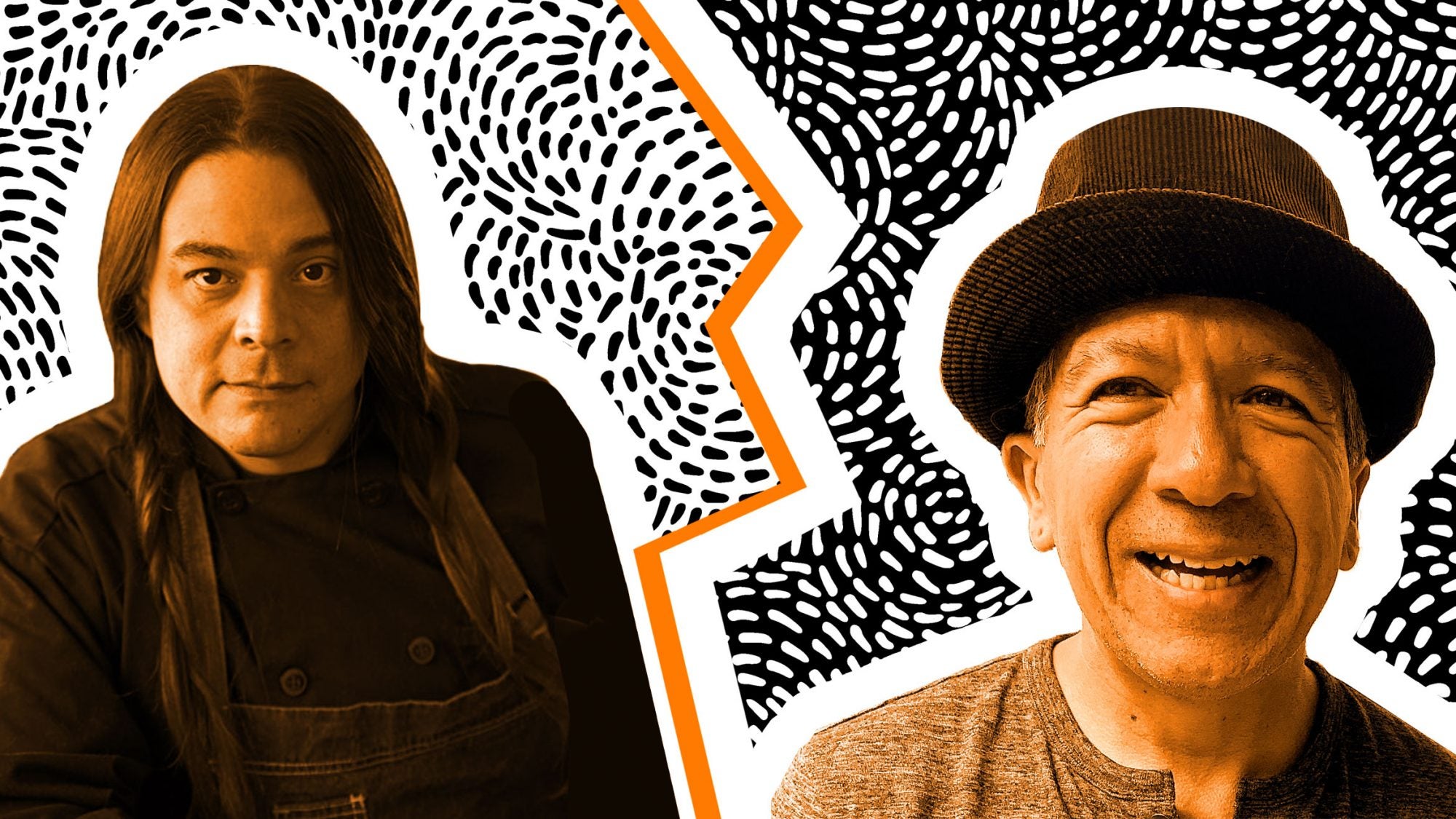This is an artsy photograph of two men with a unique, black and white design featuring an orange and yellowish-gold lightning strike-like border that separates their faces. The man on the left appears to be in his late thirties or early forties and has long dark hair styled into braided pigtails, parted in the middle. He wears black overalls with a matching long-sleeved shirt and has piercing brown eyes with a blank expression. In contrast, the man on the right, who looks to be in his mid-forties to fifties, wears a black hat and a gray t-shirt. He has a cheerful demeanor, marked by a prominent grin and a freckle on his neck. The background outlines their heads, giving the impression they have been superimposed into the image.